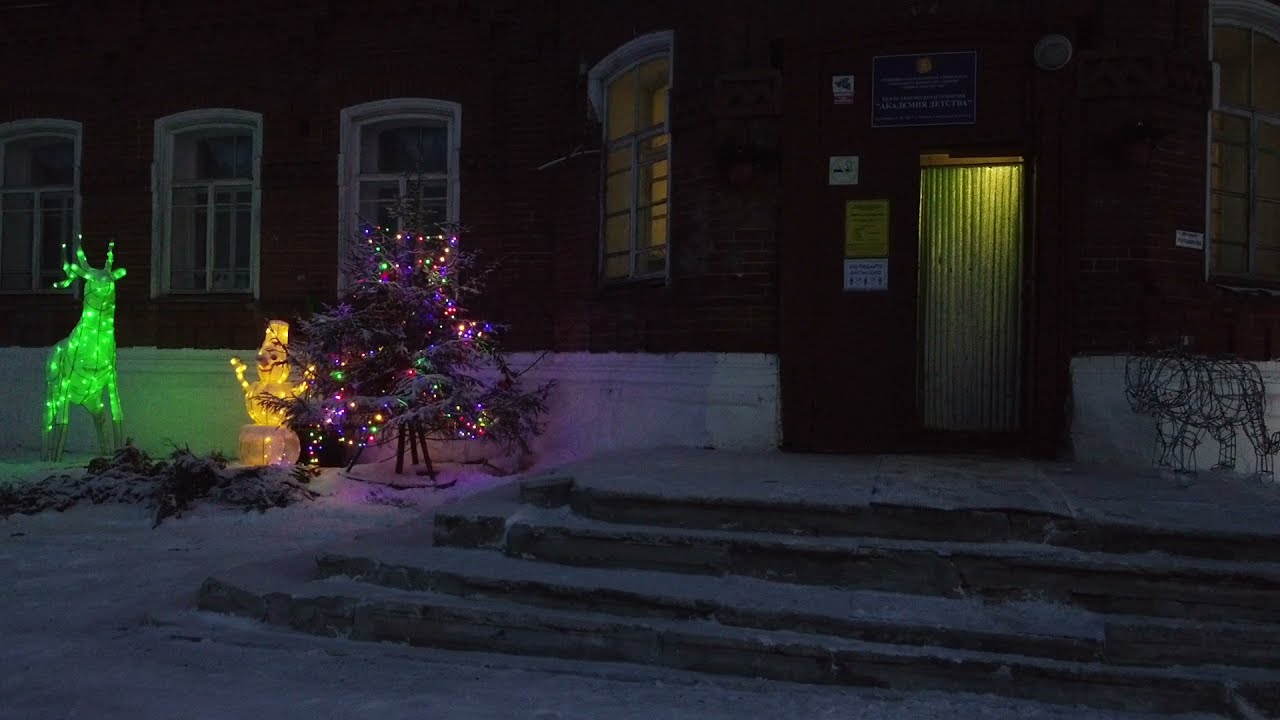This is a detailed nighttime photograph of the exterior of an older brick residential building, covered in a layer of snow. The building features white-trimmed windows and multiple signs near the entrance, including a "No Smoking" sign and one indicating surveillance. Centered on the right side is a rectangular illuminated doorway accessible by around five steps, hinting at a welcoming, light-filled interior. To the left of the entrance, a festive display celebrates Christmas, featuring a small tree adorned with multi-colored lights, a snowman glowing with yellow lights, and a reindeer lit with bright green lights. This cheerful holiday tableau, set against the backdrop of snow-covered ground and highlighted by the warm glow of decorations, reinforces the wintery, festive ambiance.